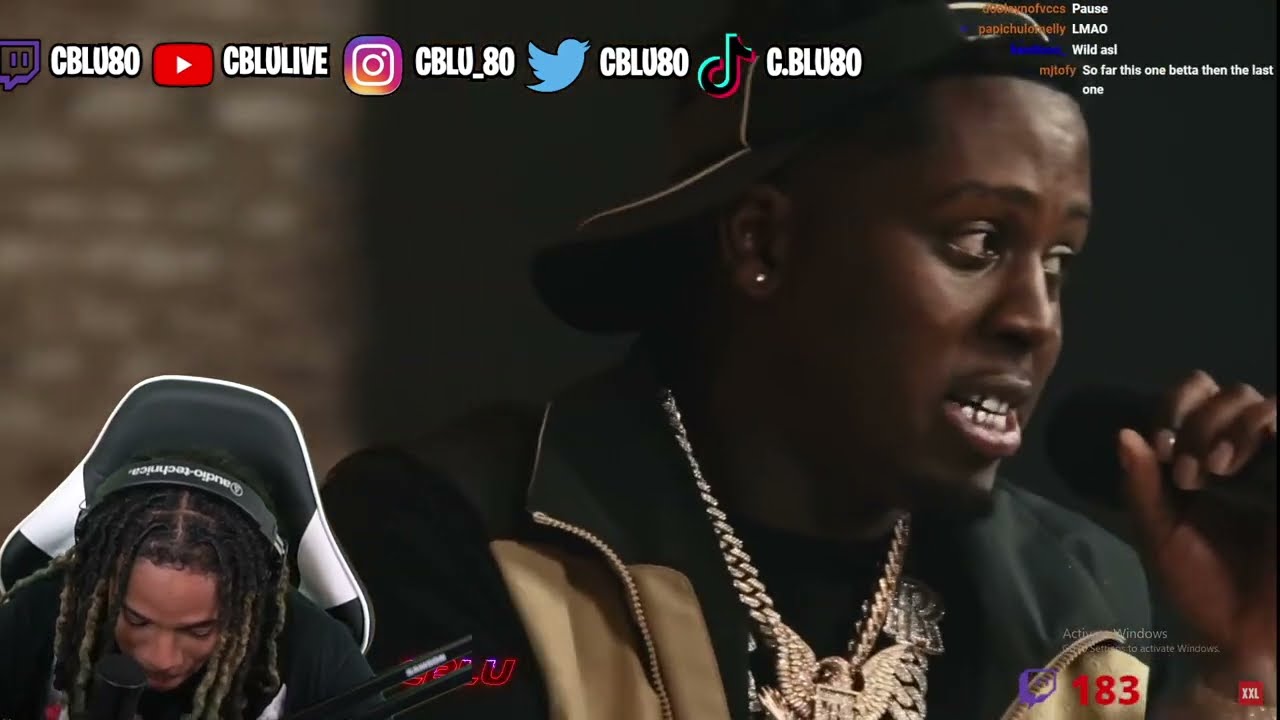The image is a detailed, colorful screenshot from an Instagram live video, possibly a podcast. Centered in the frame is an African American man, wearing a backwards baseball cap, appearing to speak mid-sentence and looking slightly to the left. In the bottom left corner, another man with dreadlocks sits in a black and white gaming chair, seemingly engrossed in watching a screen and reacting with laughter. At the top of the image, a banner displays social media tags, including YouTube (CBLULive), Instagram (see blue underscore 80), Twitter (see blue 80), and TikTok (C.blue 80). In the upper right corner, a chat box displays live viewer comments. Additionally, a Twitch logo with the number 183 in red, and a small "XXL" logo with white letters on a red background are visible at the bottom right of the image.